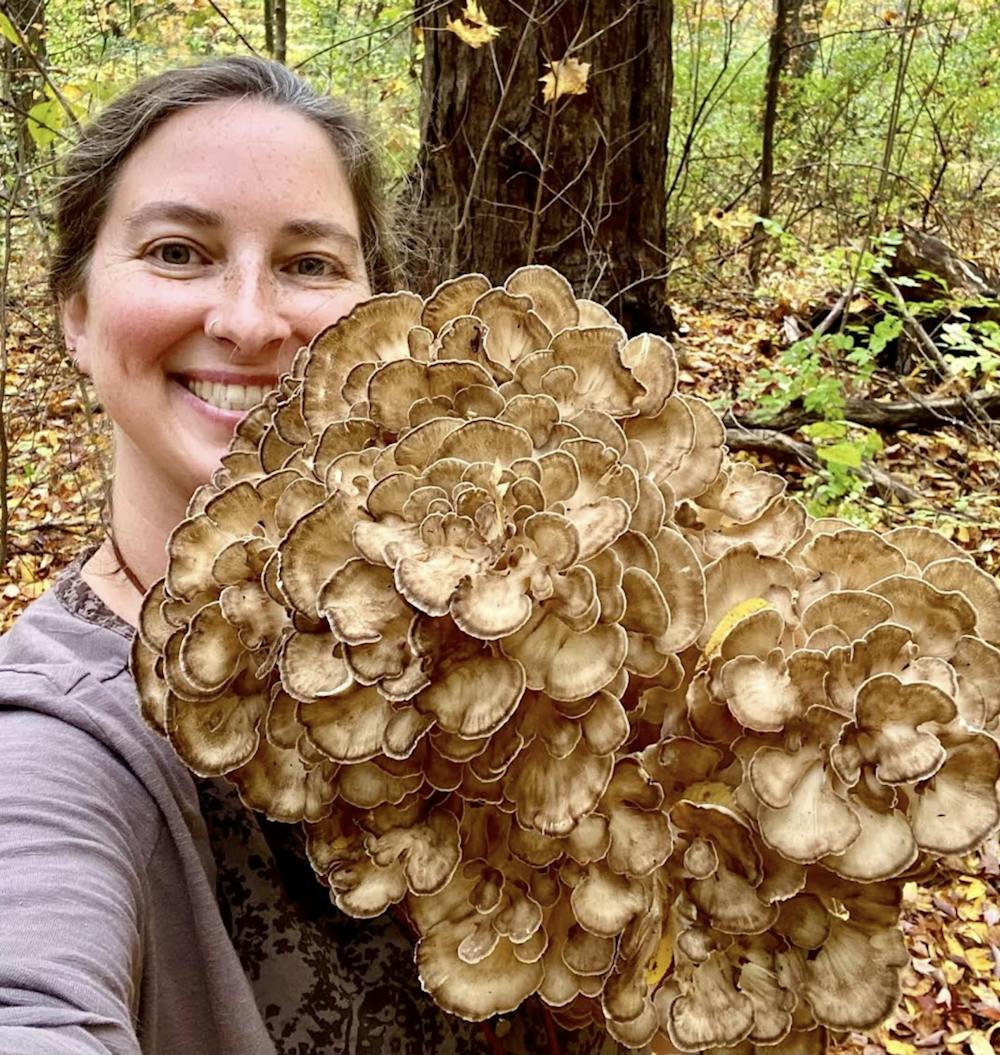In a serene woodland setting, a young woman is captured smiling brightly as she holds up an impressive, large, and intricate mushroom. The fungi, possibly a singular specimen, features multiple layered, petal-like formations with predominantly light brown hues accented by darker brown edges and occasional hints of yellow, especially noticeable on the right side. The mushroom's unique, almost floral appearance draws immediate attention.

The woman, who has light brown hair with a sprinkle of gray, wears her hair pulled back. Her face is adorned with freckles, most prominently around her nose. She is dressed in a cozy, gray long-sleeve shirt with a darker gray undershirt or scarf featuring black text or designs peeking out. There is also a hint of a brown necklace, or perhaps it's just a few strands of hair. 

In the background, there is a thick-trunked tree surrounded by smaller trees and a forest floor carpeted in dead leaves with a scattering of green ones on plants to the right. Despite the close-up nature of the photograph, the dense forest ambiance is palpable. The main colors in the image consist of various shades of brown, tan, gray, black, and touches of green, enhancing the natural and earthy vibes of the scene.